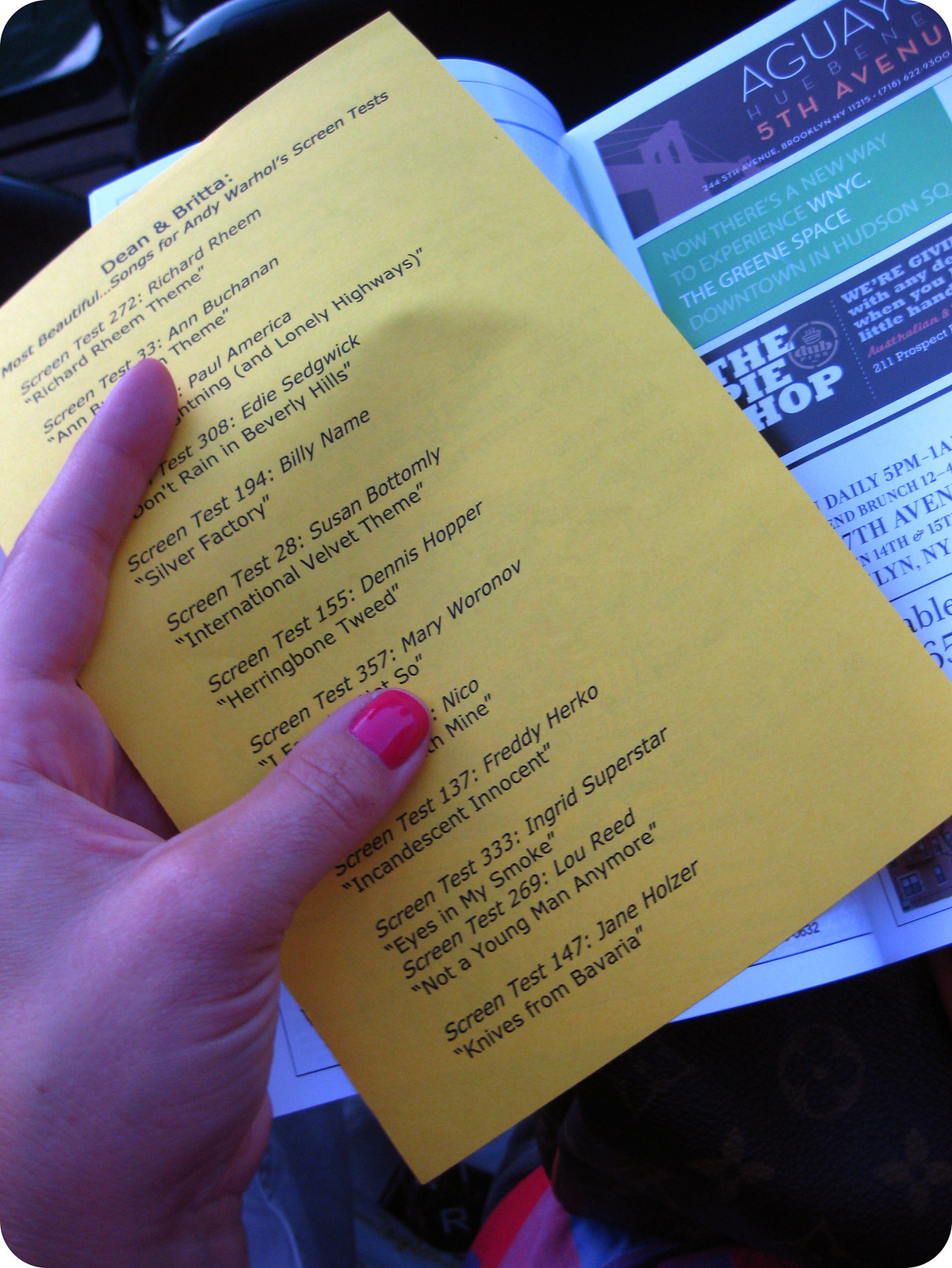In the photograph, a woman's left hand, adorned with pink nail polish, holds up a yellow 5 by 7 piece of paper prominently displaying the title "Dean and Brita: Most Beautiful Songs for Andy Warhol's Screen Test." The paper lists various screen tests with corresponding numbers and titles: "Screen Test 272," "Screen Test 194," "Screen Test 308," "Screen Test 35," "Screen Test 155," "Screen Test 357," "Screen Test 137," "Screen Test 333," and "Screen Test 147." Each screen test is detailed with specific names and descriptions, such as Richard Rheem, Paul America, Billy Name, Susan Bottomly, Dennis Hopper, Mary Woronov, Nico, Freddy Herko, Ingrid Superstar, Lou Reed, and Jane Holzer. Behind this yellow paper, more papers are partially visible, one of which is a blue pamphlet featuring the logo of the Brooklyn Bridge and text related to various New York locations and events. The setting appears to be a daytime scene, possibly indoors, with additional papers and a chair in the background. The photograph is tightly framed, focusing solely on the hand holding the paper, with no other individuals present.